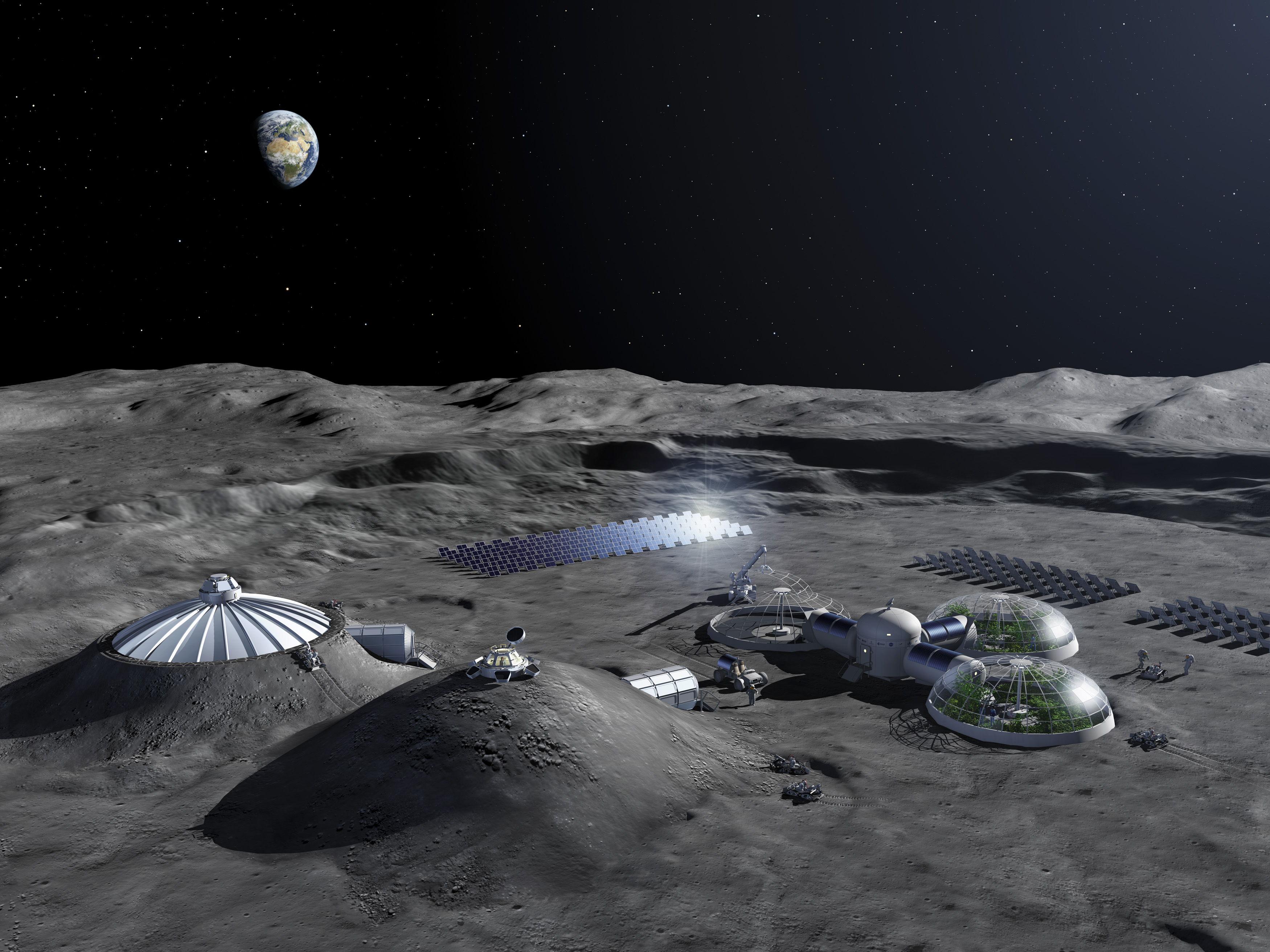The image captures a futuristic settlement on the moon against the backdrop of outer space. The rugged, gray, and cratered lunar surface is peppered with various domes and structures integrated into the mountainous terrain. Prominently, two domes feature lush greenery, visible through transparent roofs, suggesting greenhouse habitats. Scattered around the settlement are numerous solar panels, likely harnessing energy for the facility. Several vehicles, possibly solar-powered, dot the landscape, hinting at human activity. The dark expanse of space forms the backdrop, punctuated by distant stars, while Earth, partially illuminated and shrouded in shadow, occupies the upper left corner of the image. Overall, the scene portrays an advanced lunar base bathed in hues of black, gray, silver, with subtle hints of blue and brown, blending seamlessly with its extraterrestrial setting.